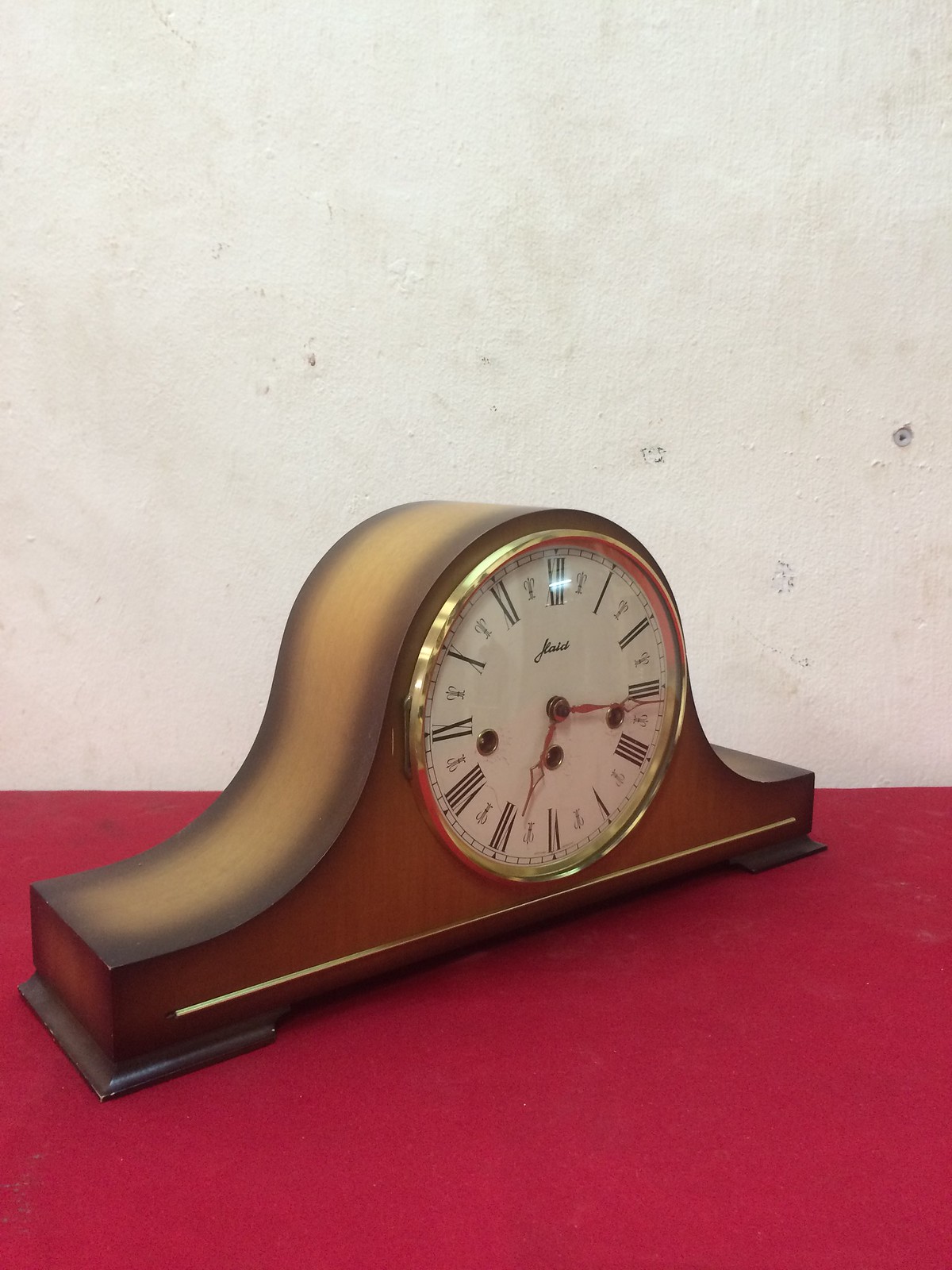This is a close-up color photograph of an antique mantle clock displayed indoors. The clock, characterized by its unique curved wooden casing, starts as a rectangle, then arches up into a near-circle before descending back down, creating a shape reminiscent of a large hump. The clock boasts a light brown front with darker chocolate brown accents on its left and right edges. However, these darker edges appear worn or sanded, giving way to a milk chocolate hue in places. A gold accent frames the white clock face, which features cursive writing at its center that is difficult to discern. The hands of the clock are silver (or possibly gold), and three small silver-lined holes are present, likely for winding the clock. The clock face displays black Roman numerals, with “XII” marking the 12 o'clock position. The background is a beat-up white wall marred with pits, black marks, and residual screw holes, suggesting the wall has been patched up multiple times. The clock rests on a maroon red felt-topped counter, adding a rich color contrast to the overall scene. The image captures a moment frozen at approximately 3:34.